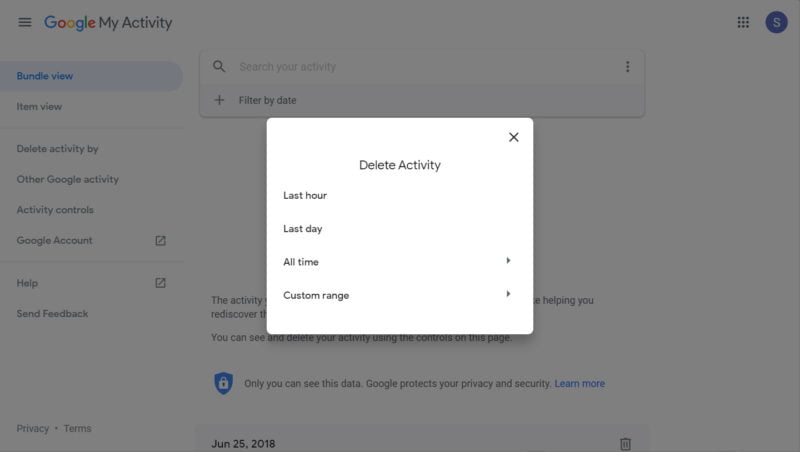The image is a horizontally rectangular screenshot from the Google My Activity page. The page itself has a gray overlay, indicating that a pop-up window is active. In the center of the screen, a white pop-up square is displayed. This pop-up has an "X" in the top right corner to close it. Centrally, the text "Delete Activity" is prominently featured. Below, there is a left-aligned list of options, including "Last Hour," "Last Day," and "All Time," each accompanied by a forward arrow. Additionally, a "Custom Range" option is listed, also with a forward arrow beside it.

Behind the gray overlay, the main Google My Activity page can be seen. At the top left corner, the Google logo is displayed, followed by the "My Activity" text. Directly beneath, there is a vertical menu with several options: "Bundle View" (highlighted in blue), "Item View," "Delete Activity By," "Other Google Activity Controls," "Google Account," "Help," and "Send Feedback." 

In the central top section of the main page, just below the header, there is a search text window labeled "Search your activity," accompanied by a "Filter by date" option.

Beneath the white pop-up window, in the faintly visible main page background, there is a message: "Only you can see this data. Google protects your privacy and security," followed by a "Learn more" link in blue.